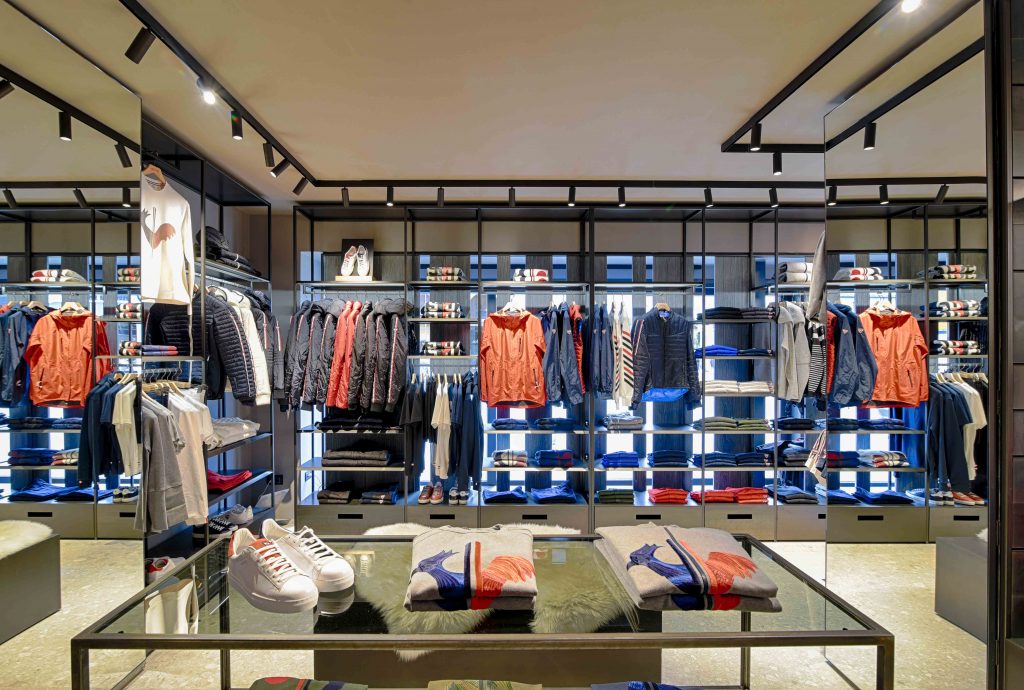The photograph portrays a high-end men's clothing store with an organized and stylish layout. The floor has a greenish-beige hue that complements the beige ceiling, which features a black track with small cylindrical light fixtures strategically angled to illuminate the merchandise. The back wall is grey, adorned with shelves that have a grey base and light silvery tops. These shelves are laden with folded clothing items and display jackets. On the left-hand upper shelf, white shoes are showcased in a black box, with more folded clothes adjacent to them. Two vertical mirrors on the left and right sides of the frame reflect this scene, adding depth to the image.

Centrally positioned at the bottom of the frame is a glass table with a sleek metal structure, presenting a pair of white shoes on the left and a folded grey shirt with a vibrant bird design—the bird featuring an orange right side and a blue left side. A stack of similar shirts lies to the right. The store exudes a sophisticated atmosphere, highlighted by the varied colors—orange, black, blue, white, dark navy, and melon—of the clothing items, which include a mix of jackets, shirts, and shoes. Track lighting on the ceiling enhances the display, making the fashionable garments stand out.